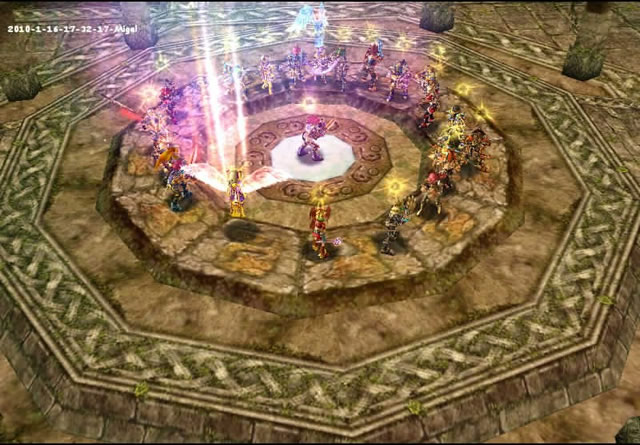This detailed screenshot captures a moment in a massively multiplayer online (MMO) game, set in what appears to be an ancient, stone-crafted temple intricately designed with multiple concentric circles. The outermost ring features an elaborate rope-like pattern, masterfully carved from stone and adorned with patches of green moss or algae, adding a touch of nature to the otherwise rigid structure.

An inner ring, composed of larger stones arranged in a perfect circle, acts as a platform for numerous players. They stand evenly spaced around the perimeter of this ring, creating a striking formation. At the core of this assembly lies another decorative circle, intricately designed and serving as the focal point of the scene. Positioned at the very center of this innermost circle is a single player, surrounded by the disciplined formation of their fellow gamers, suggesting a ceremonial or significant event within this virtual world.